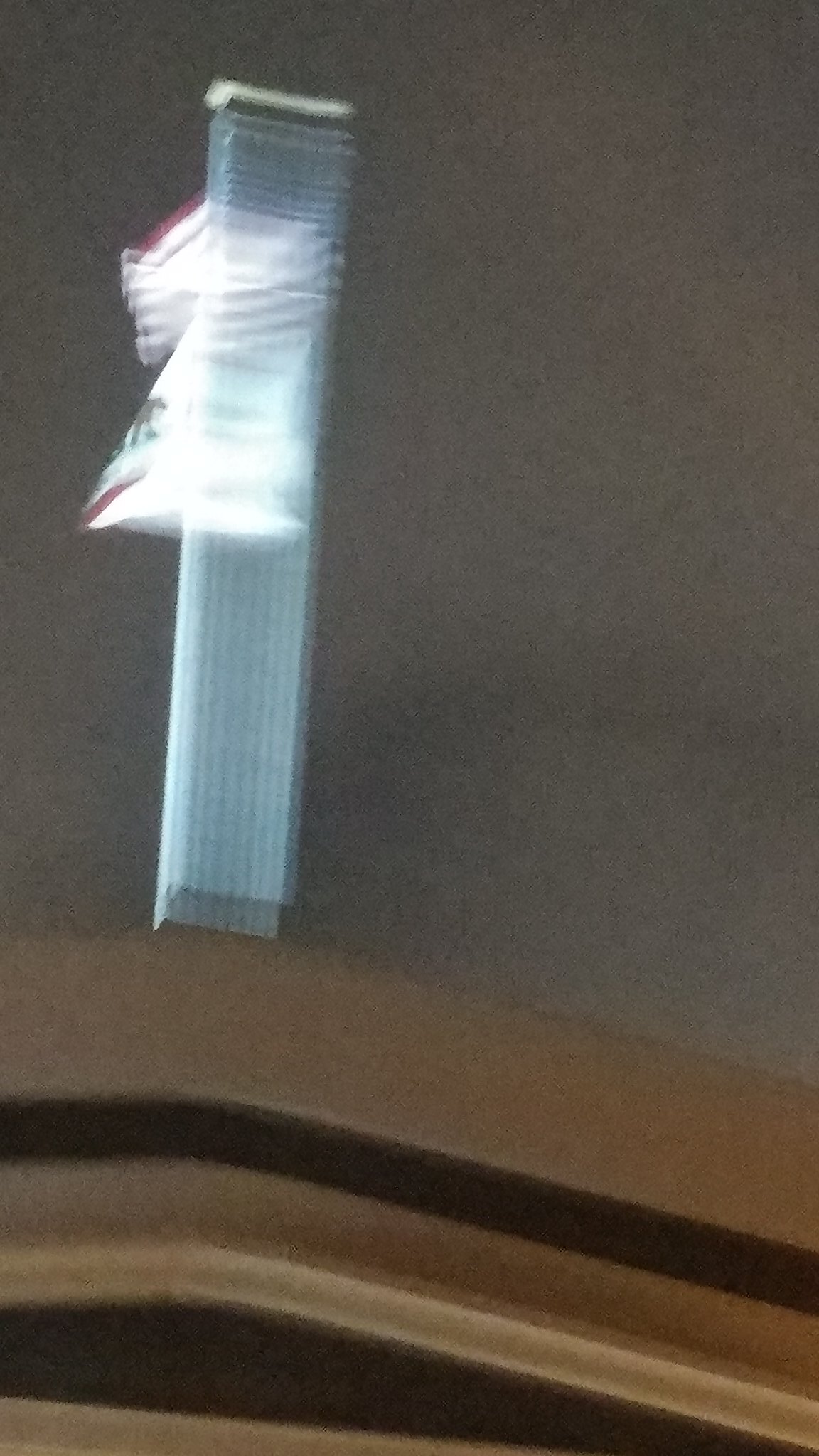In the image, the background is predominantly dark brown. On the left side, a tall, thick bar in a vivid blue color rises vertically. Intriguingly, the center of this blue bar is illuminated by a white light, which is bordered at the top with a red trim. At the very top of the image, the blue bar merges with a white section. Below this, a broad horizontal bar of dark brown spans across the composition. Underneath, there is an extensive area of very dark brown, followed by a sequence of color bands transitioning from dark brown to a lighter brown stripe, and then back to a medium brown shade. The image's structure and color palette create a layered visual effect, with the interplay of blues and browns capturing the eye. The purpose or subject matter of the image remains ambiguous, adding an element of intrigue.